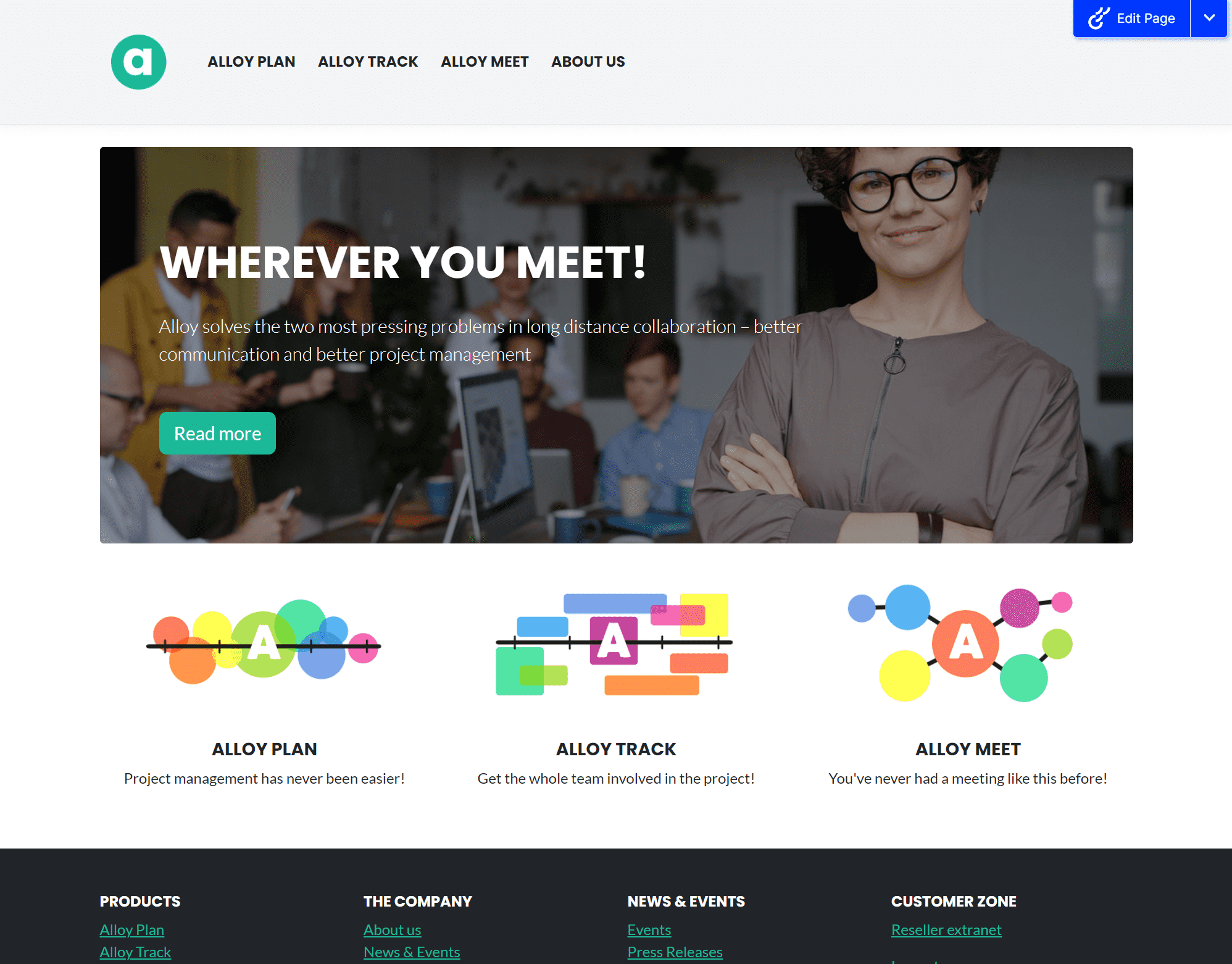**Detailed Caption:**

The screenshot features a modern website layout with a light gray rectangular navigation bar at the top. On the left side of this bar, there is a green circle containing a white lowercase 'a'. Adjacent to this circle, bold black text displays the words "Alloy Plan", "Alloy Track", and "Alloy Meet". Further to the right, centered on the top of the page, "About Us" is also written in bold black letters.

On the far right end of the navigation bar, there is a blue button featuring an image of white chain links on the left side and the text "Edit Page" in white. Next to the button, a downward-facing white arrow resides within a blue box, indicating a dropdown menu.

Descending to the main content area, a background image features a group of people sitting around a table, each with coffee cups in front of them. On the left, a man in a yellow shirt with a white undershirt holds a coffee cup. To his right, a woman with shoulder-length red hair dons a black dress while also holding a coffee cup. Two men sit on the floor to the right, focused on a silver laptop; the man on the right has short dark hair and wears a brown shirt, while the man on the left has short brown hair, pale skin, and a long-sleeved blue shirt.

Foregrounded on the left, bold white text reads, "Wherever you meet," followed by a smaller caption stating, "Alloy solves the two most pressing problems in long distance collaboration: better communication and better project management." Below this text, a teal button with white text reads, "Read More".

To the right in the foreground, a woman with short, curly brown hair, pale skin, and black circular-rimmed glasses is distinguished by her tan zip-up long sleeve shirt.

Beneath this section, a white rectangular area showcases three distinct icons left to right: the first is a black line with horizontal and vertical details, surrounded by bubbles of various colors (red, orange, yellow, green, teal, blue, and purple), and features a white capital 'A' at its center. The second icon, similar in structure, has multi-colored stripes and is encased in a purple box. The third icon resembles a sideways 'X' with colored bubbles passing through it, centered around a peach-colored circle with a white capital 'A'.

Below these icons, three sections provide additional details:

- **Alloy Plan:** "Project management has never been easier."
- **Alloy Track:** "Get the whole team involved in the project."
- **Alloy Meet:** "You've never had a meeting like this before."

At the bottom, a black bar contains four white menu headings. 

- **Products:** Sub-options "Alloy Plan" and "Alloy Track" are listed in blue.
- **The Company:** Sub-options "About Us" and "News and Events" are in blue.
- **News and Events:** Sub-options include “Events” and “Press releases,” both listed in blue.
- **Customer Zone:** Featuring "Reseller Extra Net" below in blue bold text.

The bottommost area of the screenshot appears to be cut off.